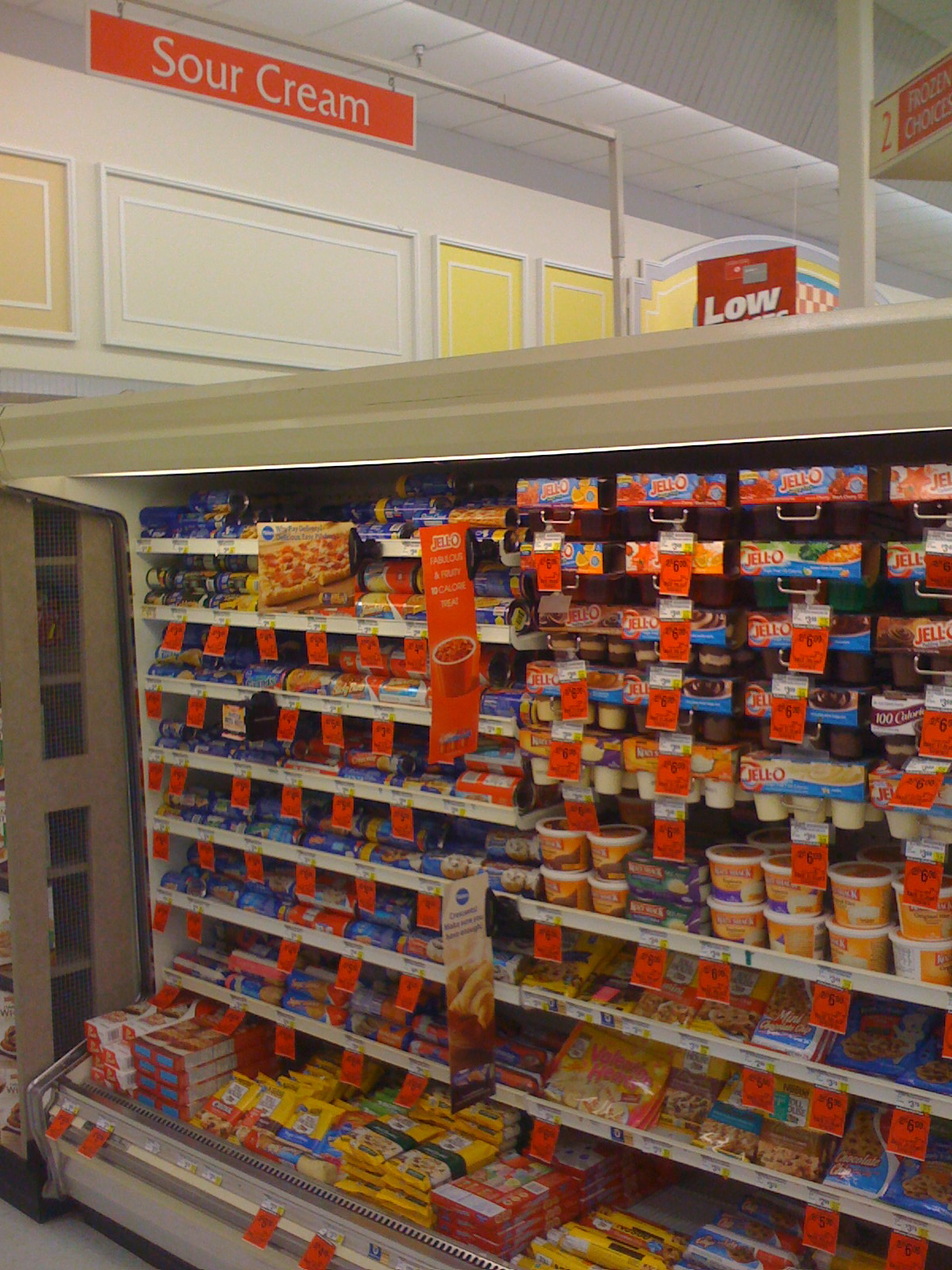A close-up photograph captures a section of an open refrigerator in a supermarket, specifically the area displaying a vast array of yogurts and jellos. The scene is meticulously organized, with the products neatly aligned in approximately seven or eight rows across two separate bays. Visible price tags adorn each item, some highlighted with orange stickers likely indicating discounts. The angle of the shot reveals not only the pristine display case but also a glimpse of the supermarket’s ceiling and part of the floor at the bottom of the image. Additionally, overhead signage marking sections for sour cream and frozen items punctuates the background, providing context to the location within the store. The overall impression is one of orderliness and a well-stocked dairy and dessert section.